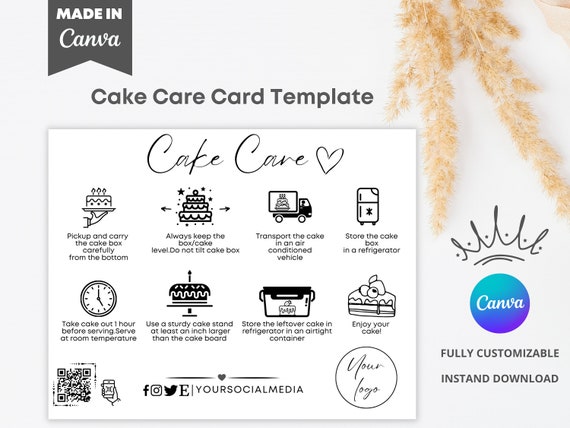The image illustrates a detailed Cake Care Card Template made using Canva, prominently labeled "Made in Canva" in the top left. The main content of the template includes a header "Cake Care" accompanied by a small heart icon, followed by a two-row, four-column grid detailing cake handling and storage instructions. The instructions read: "Pick up and carry the cake box carefully from the bottom; Always keep the box/cake level; Do not tilt cake box; Transport the cake in an air-conditioned vehicle; Store the cake box in a refrigerator; Take cake out one hour before serving; Serve at room temperature; Use a sturdy cake stand at least an inch larger than the cake board; Store the leftover cake in a refrigerator in an airtight container; Enjoy your cake." Icons representing cakes and slices enhance the instructions. A QR code is located in the bottom left corner, alongside logos for social media platforms like Facebook, Instagram, Twitter, and Etsy. The bottom right corner features a customizable logo area labeled "Your Logo," and states "Fully customizable, instant download" in black font. The border of the whole image includes a decorative element depicting wheat in the top right corner.